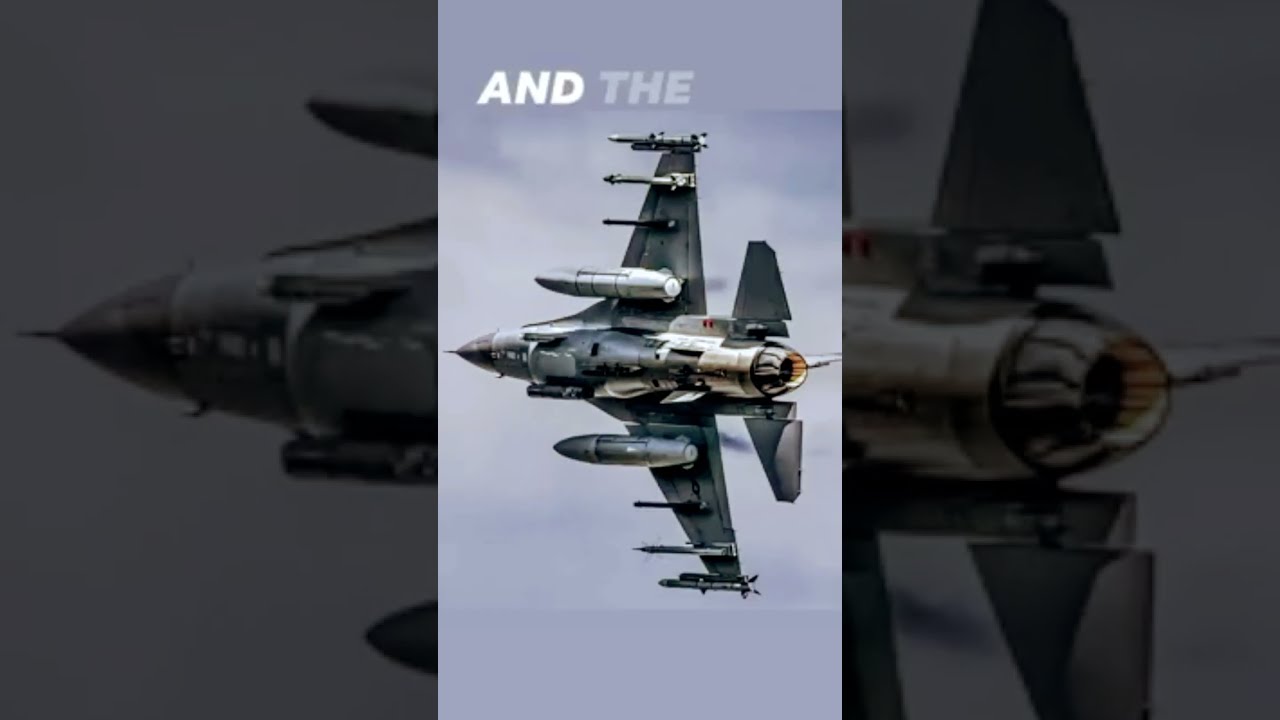The image is a three-panel photograph with the left and right panels darkened out, emphasizing the brightly lit center panel. In this central, portrait-oriented image, we see the underside of a grayish fighter jet flying horizontally at a 90-degree angle. The jet's bottom is clearly visible, adorned with six smaller rockets—three on each wing—and two larger missiles near the body. The sky blue background contrasts with the jet's detailed underbelly and the streamlined, needle-point front. The jet has an aqua-ish blue tint on its wings and flaps, adding to the visual appeal. Above the jet, the text reads "and the."